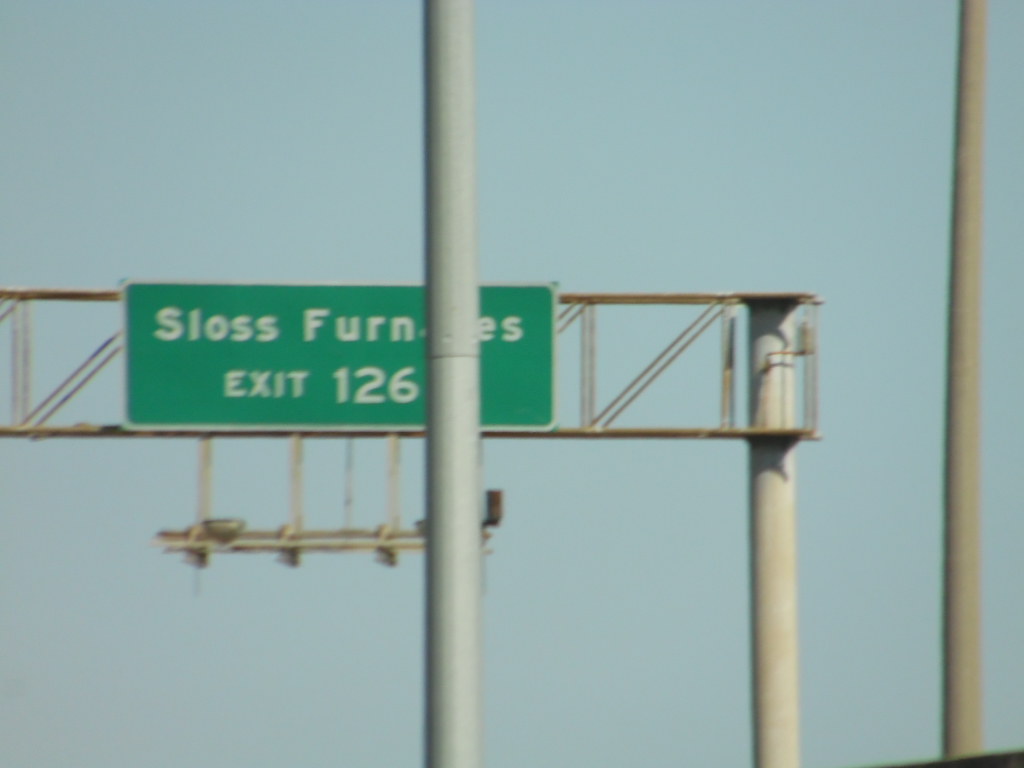Daytime outdoor image of a traffic sign supported by multiple steel gray poles. The far-right pole extends from the bottom of the frame and continues past the top, while the central pole holds up the traffic sign. An additional pole is situated directly in front of the sign, partly obscuring it. The sign itself is a long green rectangle with white text. It appears to read "SLOS FURNACES", though the pole blocks part of the text, leaving only "SLOS FERN, F-U-R-N," and an "E" followed by an "S" visible. Below the main text, it indicates "Exit 126." Behind the sign, scaffolding in intermittent V shapes supports the structure.